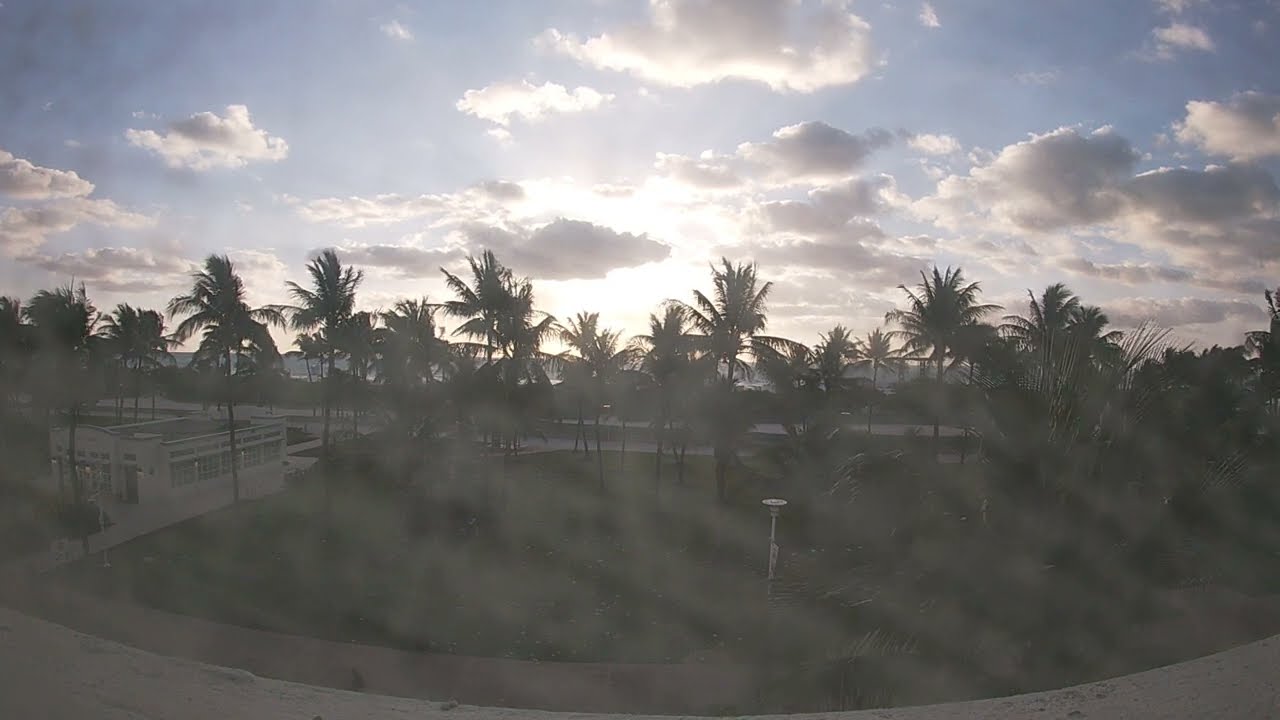The image captures an outdoor scene dominated by numerous palm trees stretching across the entire view from left to right. The sky occupies a substantial portion at the top, filled with large, fluffy white clouds partially obscuring the sun, which bathes the scene in natural light indicative of daytime. The overall image is very blurry, creating an impression of shadows and indistinct forms. On the left edge, a white building or small facility is partially visible. In the background, roads can be vaguely discerned. The setting is devoid of people and vehicles, featuring only the palm trees, distant roads, and ample grass amidst a haze of unclear details.